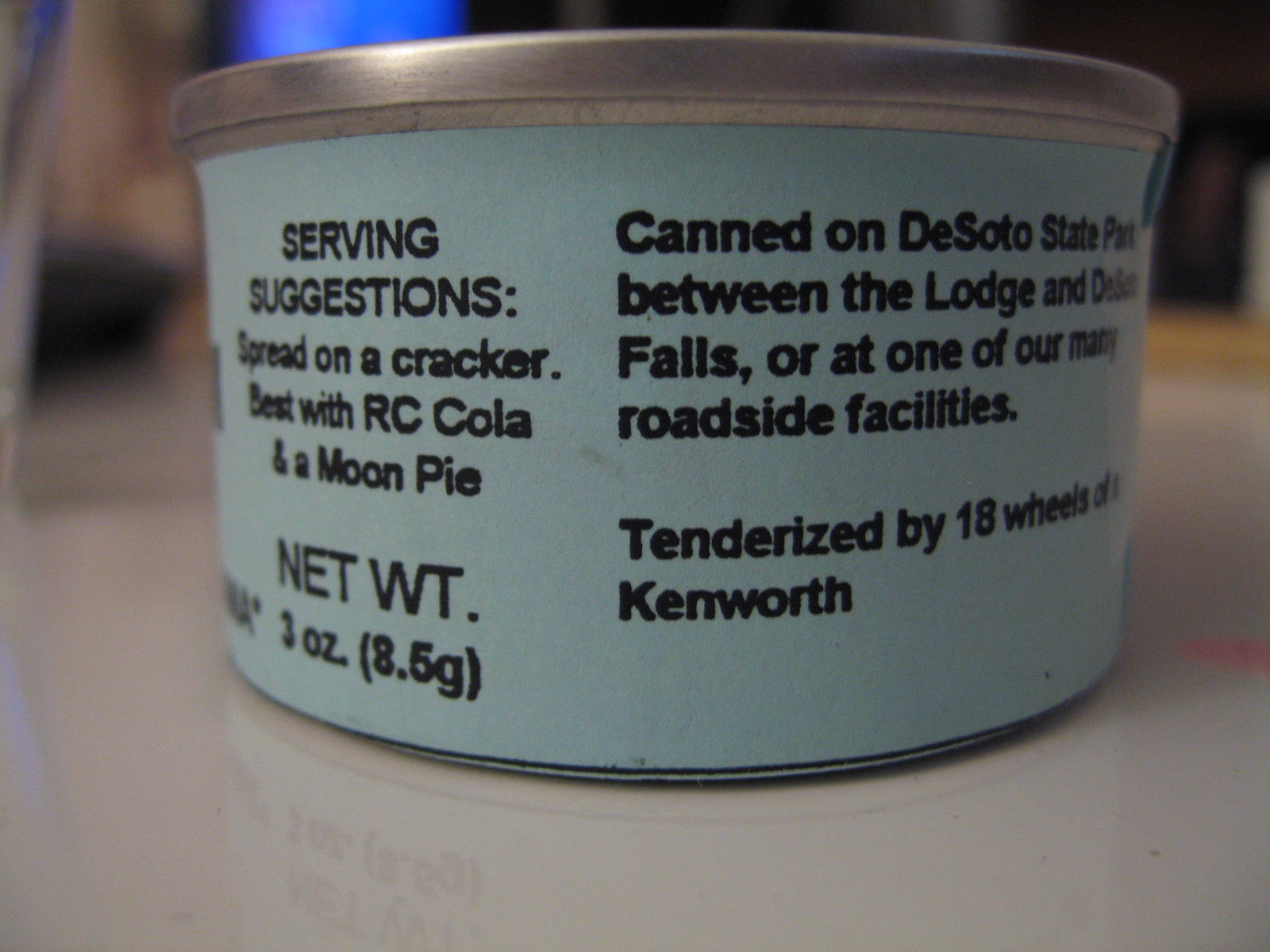In this close-up image, we see a peculiar can occupying most of the frame, positioned on a white table. The can itself is white with contrasting black lettering and features a silver metallic top. The foreground text details serving suggestions, recommending the spread be enjoyed on a cracker, complemented by RC Cola and a Moon Pie. It also lists the net weight as 3 ounces (8.5 grams). Additional text on the right-hand side indicates the spread was "canned at DeSoto State Park, between the lodge and DeSoto Falls, or at one of our many roadside facilities," and intriguingly notes it was "tenderized by 18 wheels of Kenworth." The background is blurred with indistinct patches of blue, black, and yellow, providing no further context and ensuring the can is the focal point of the image.